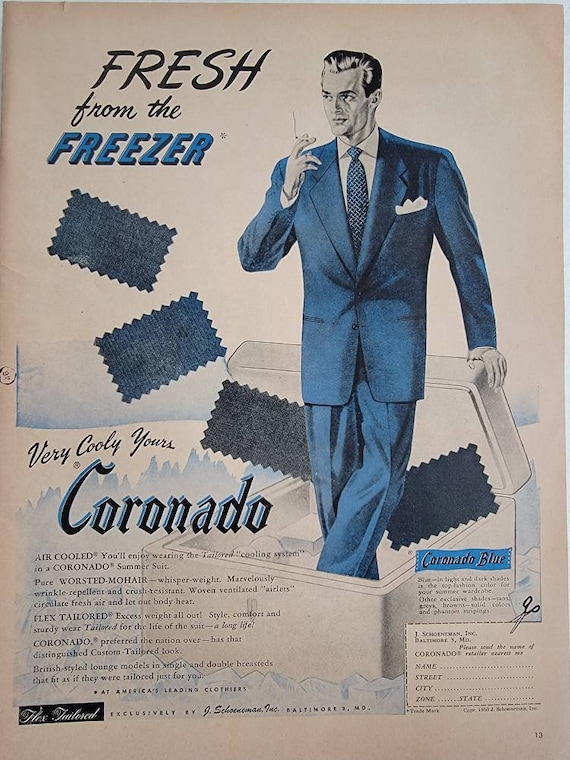The image depicts a vintage magazine advertisement for the "Coronado" men's suit, characterized by a slightly worn and weathered page. On the right side of the image stands a sketched gentleman, prominently centered in the page, wearing a blue suit complete with a blue tie, a white button-down shirt, and a white handkerchief in his upper pocket. He has black coiffed hair and is smoking a cigarette with his right hand, while his left arm rests on the lid of a large, white freezer chest in which he is standing.

Swatches of different blue fabrics fly out from the opened chest, and below them lays a bed of ice cubes and mini mountains, adding to the coolness theme. The top of the ad features text in a mix of black and blue font that reads, "Fresh from the freezer, very coolly yours, Coronado Blue." Detailed information about the suit is stated in three text paragraphs, highlighting features like "air-cooled, worsted mohair" and "flex tailored." The coupon box in the lower right corner includes a set of scissors icon and fields for name and address, directing submissions to Jay Schonman Incorporated in Baltimore, Maryland. At the bottom, the text proudly proclaims the suit as "fine tailored exclusively by Jay Schonman Incorporated" and touts the cool Coronado suit.